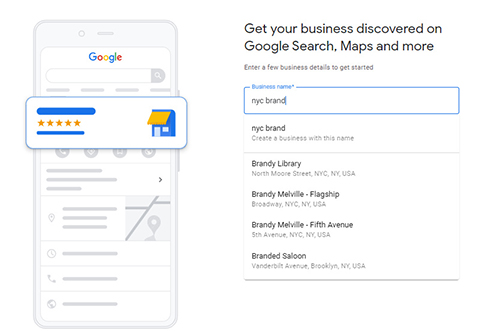A screenshot detailing instructions for enhancing the visibility of a Google Business profile on Google Search. The background is entirely white. On the left side, an image of a mobile phone displays the Google interface, featuring the Google logo at the top. Below, there's a business icon accompanied by a section showing five yellow stars, indicative of customer reviews. An image of a house is also present.

On the right, bold text instructs viewers on how to get their business discovered across Google Search, Maps, and other platforms. It encourages entering free business details to begin. In the search box, an example query "NYC brand" is shown. Subsequent search results suggest options such as Brandy Library, Brandy Melville, and Branded Salon, indicating the system's prompts for related businesses.